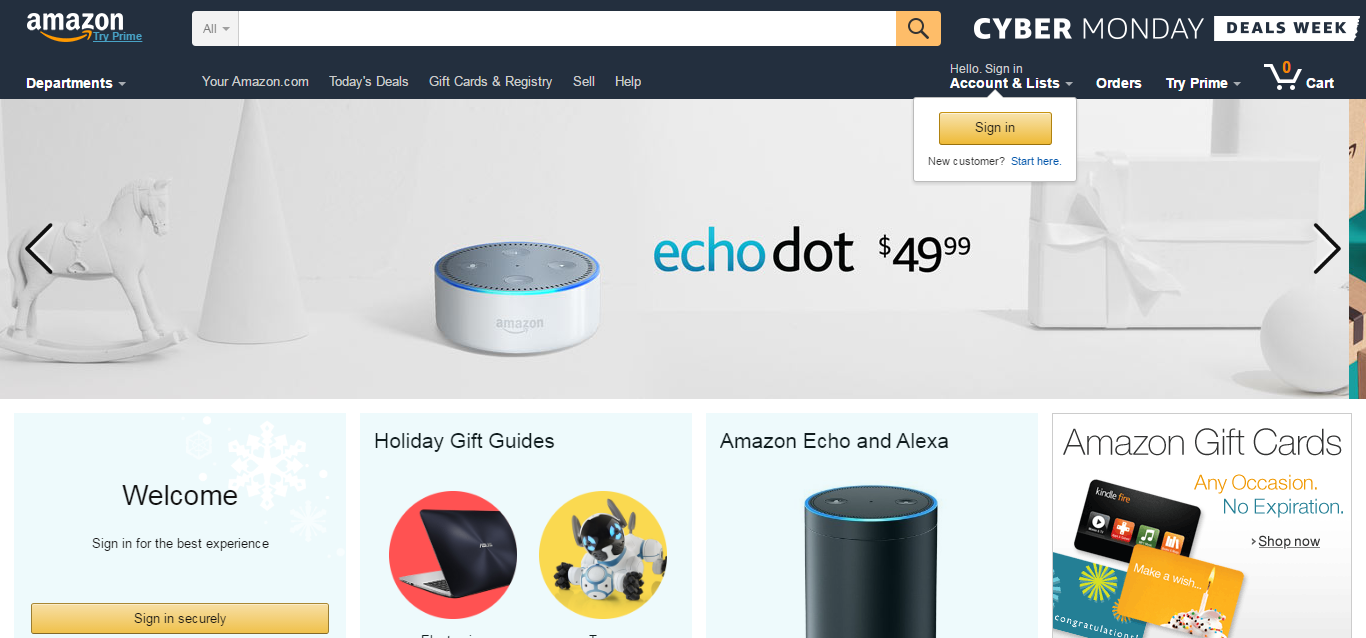The image displays the desktop version of the Amazon website. The top 15-20% of the screen is dominated by a dark blue navigation bar. On the far left of this bar, the iconic Amazon logo is prominently featured in white with the characteristic orange arrow pointing from 'A' to 'Z'. Beneath the logo, there is a blue hyperlink labeled "Try Prime."

To the right of this, a large search box spans across much of the bar, followed by an orange search button with a black magnifying glass icon. Immediately to the right of the search button, a blue text advertises "Cyber Monday Deals Week."

Moving further right on the navigation bar, there is a dropdown menu for browsing "Departments," which is currently selected. Adjacent to this menu, you'll find several links: "Your Amazon.com," "Today's Deals," "Gift Cards & Registries," "Sell," and "Help."

Shifting to the far right section of the bar, the text "Hello, Sign In, Accounts & Lists" invites users to log in. Below this prompt, an orange button labeled "Sign In" is displayed, followed by the text "New customer? Start here" in blue. Next to these login options are additional links for "Orders," "Try Prime," and "Cart," which features a shopping cart icon with an orange zero, indicating an empty cart.

Below this navigation bar, the main content area begins, taking up approximately half of the page with a promotion banner for the Echo Dot priced at $49.99. The banner includes an image of the Echo Dot on the left, while an illustration of a rocking horse and a cone sits beside it. To the right, a package is depicted, all set against a white background.

Further down, the page is segmented into four distinct sections, each catering to different categories: "Welcome," "Holiday Gift Guides," "Amazon Echo & Alexa," and "Amazon Gift Cards." These sections are evenly divided from left to right, providing a clear and organized layout for easy navigation.